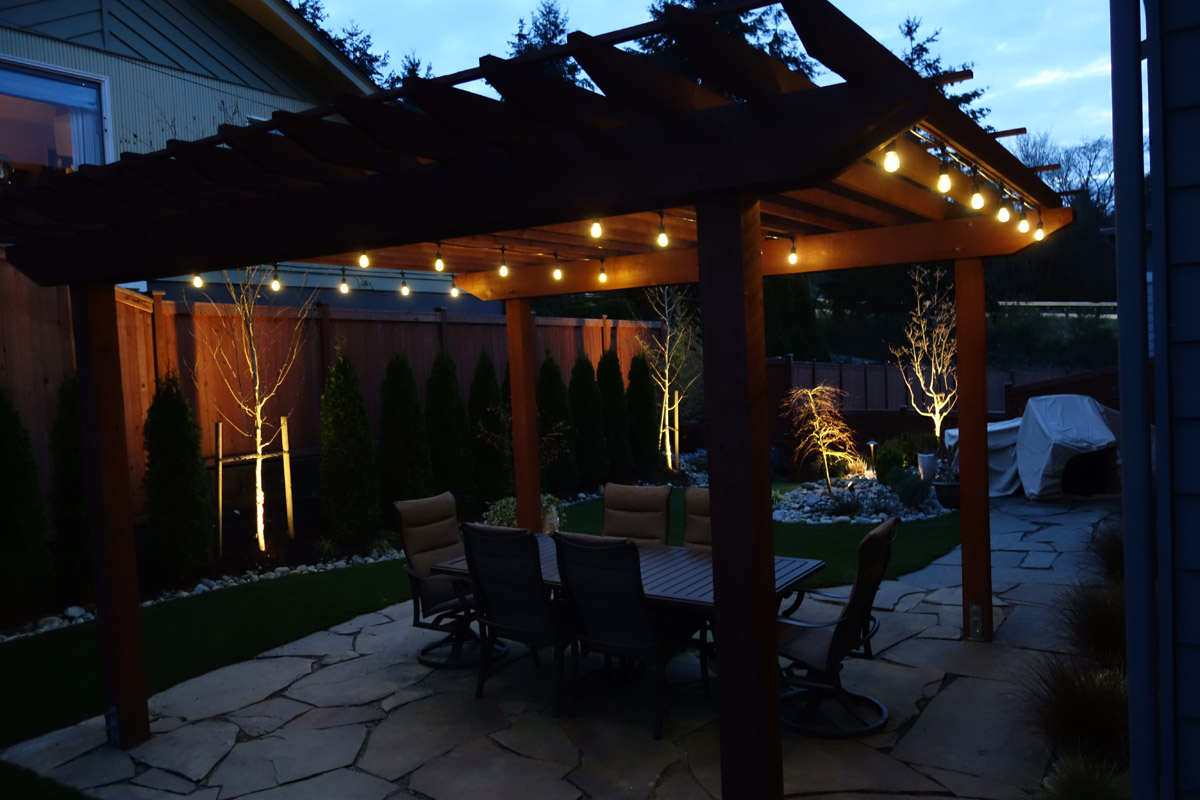The image captures a nighttime scene of a well-maintained backyard patio with distinctive Asian-inspired architecture, which appears to be an open, rectangular pavilion made of wood, resembling a pagoda or gazebo. This pavilion stands on a patio with a flagstone surface and features four substantial wooden supports. Thin wooden slats form the roof, allowing glimpses through, and numerous yellow light bulbs hang from the ceiling, providing a warm illumination in the dark, shadowed setting. Underneath the pavilion, there's a rectangular wooden table surrounded by six chairs, arranged with two at each end and two on each side.

To the left of the patio, there is a tall wooden fence separating this area from the neighboring house, behind which stands a row of decorative shrubs and skinny trees. The background reveals a mix of landscaping elements, including a large boulder, additional trees, and a grassy area, most of which are barren, suggesting perhaps an off-season or recent pruning. On the right edge of the image, a fragment of the house to which the patio belongs is visible, alongside a potential gate or wall that marks the boundary of the property. The sky above is softly illuminated in a blue hue, indicating the twilight hour, and beyond the wall, a distant railing that might border a road or sidewalk is partially seen amongst further trees, completing this picturesque and intimate outdoor space.